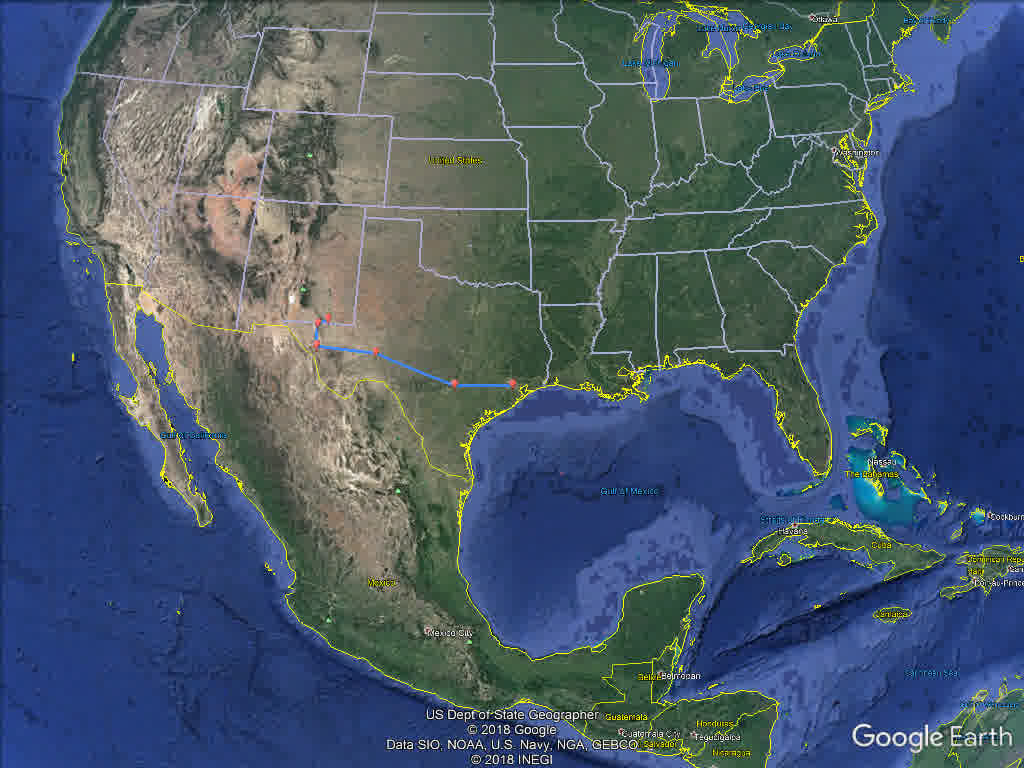This image is a screenshot from a geographic website, featuring detailed visual data. At the bottom right-hand corner, the text "Google Earth" is displayed in white font, attributing the source of the image. Centrally positioned text reads "U.S. Department of State Geography, copyright 2018 Google," indicating the image's relevancy and date of information.

The map prominently showcases the United States, with noticeable inclusion of Mexico, providing a comprehensive view of the terrain. In California and along the west coast, brown and dark gray patches denote desert regions, indicating sparse vegetation and arid conditions. The majority of the map, however, is adorned in green hues, representing areas with richer vegetation and diverse landscapes. Notably, a distinctive yellow border outlines the east coast, likely highlighting state boundaries or specific geographic features.